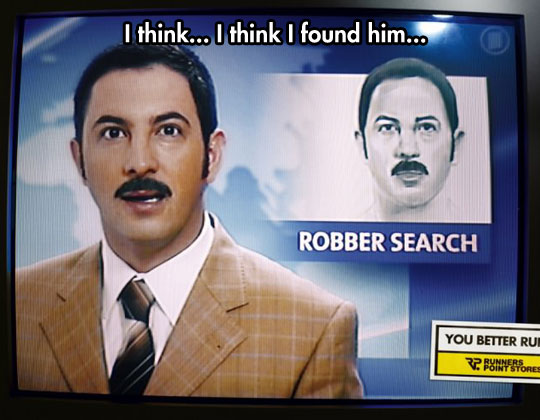This photograph appears to be a humorous meme, captured from a television screen, possibly during a newscast. The image features a news anchor with short black hair, black eyebrows, and a black mustache. He is dressed in a tan, checkered sports jacket, white shirt, and a brown tie. The text at the top of the screen reads, "I think... I think I found him..." in white letters encased in a black border. To the right of the anchor, another image, possibly a black-and-white drawing or a cropped photograph, shows a man who looks remarkably similar to the news anchor, also featuring short black hair, black eyebrows, and a mustache. Below this second image, the text reads, "Robber Search." The background consists of blue and white colors. In the lower right-hand corner of the screen, a white rectangle with vertical orientation contains the text "You Better Run" with a thick black line underneath, followed by the partially visible phrase "Runners Point Stores" in yellow. This resemblance between the newscaster and the suspect creates the comedic effect central to the meme.